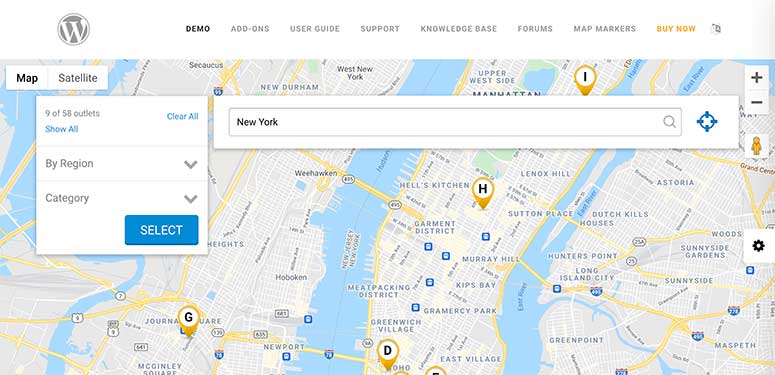This is a detailed map of a segment of New York City, accompanied by a top navigation bar containing the links: "Demo," "Add-ons," "User Guides," "Support," "Knowledge Base," "Forums," "Map Markers," and "Buy Now." Beneath this bar is a text box labeled "New York," flanked by options to switch between "Map" and "Satellite" views. It also shows "9 of 58 outlets" with categorized filter options accessible through two dropdown menus labeled "By region" and "Category," next to a blue "Select" button.

The map itself is intricately labeled with various notable neighborhoods, including Garment District, Hell's Kitchen, Lenox Hill, Manhattan, Sutton Place, Dutch Kills Houses, Astoria, Hunters Point, Long Island City, Sunnyside, Greenpoint, and East Village. Several pins are placed across the map, each marked with different letters such as G, H, and D. A number of streets are highlighted in yellow, though specific street names are sparse and significantly blurred.

The geographical scope of the map extends to show parts of New Jersey, separated by a visible boundary line from New York City. Despite its detailed context, the text labeling the streets remains difficult to read due to its blurriness. The upper left corner of the map features a circle with the letter W inside it, possibly representing some form of map marker or legend.